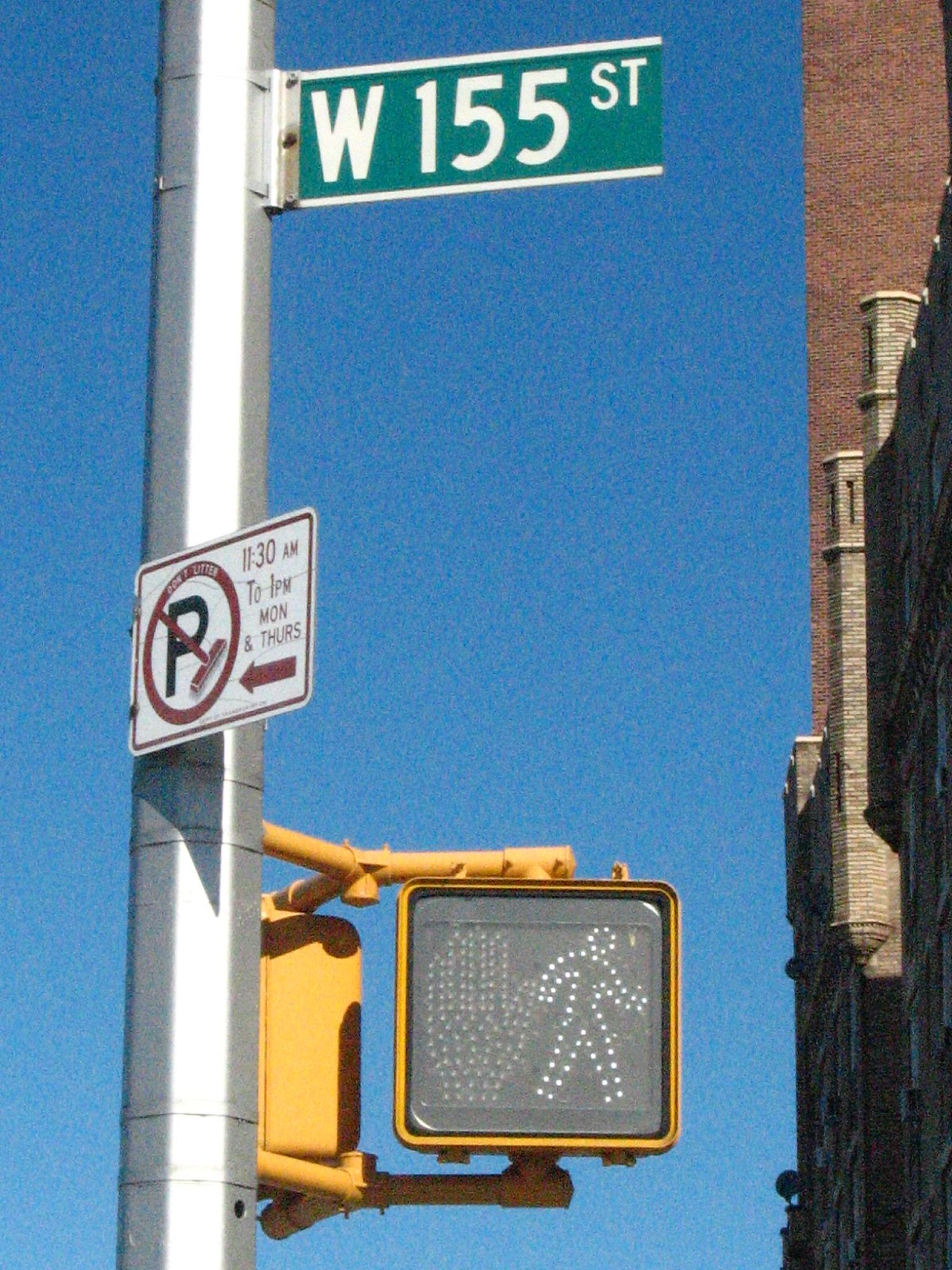A shiny, silver metal pole stands tall in this photo taken outdoors under a clear, cloudless blue sky. At the bottom of the pole is a yellow square box that houses a crosswalk signal, currently displaying a lit walking man icon, symbolizing it is safe to walk. Behind this signal, another crosswalk signal faces the opposite direction, showing a non-illuminated stop hand. Above this, a white background sign with red text and circles announces "No Parking 11:30 AM to 1 PM Monday through Thursday" and includes a left-pointing arrow. At the top of the pole, a rectangular green street sign with white lettering reads "West 155th Street." To the right of the pole, the facade of a tall building, partly brick and partly adorned with stone towers, complements the urban scene.